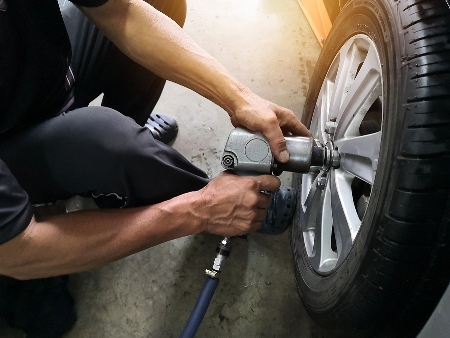In the image, a Caucasian male is depicted in the process of removing a tire from a vehicle. He is dressed in a black t-shirt, black pants, and grey shoes. Utilizing a grey metal device connected to a compressor via a blue rubberized hose, he is unscrewing the bolts from the tire. The floor beneath him is grey concrete. The tire, which is black with visible ridges, features silver bolts and a silver rim. The vehicle's body, visible at the far edge, appears to be grey. The metal device he is using to remove the bolts has a grey indented circle on its silver handle.